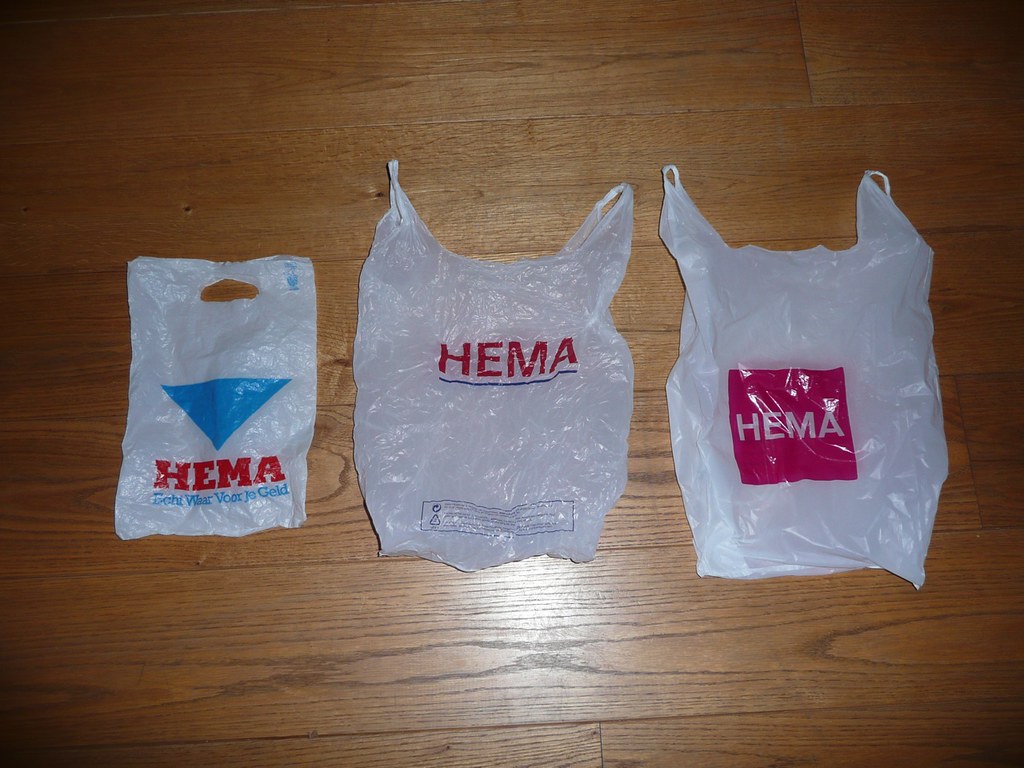The image captures a close-up scene of three plastic shopping bags arranged on a deep brown wooden floor with distinct grain patterns resembling wide, thin ovals. Centered within the frame, the bags share the common detail of featuring the word "HEMA" prominently. The bag on the left is the smallest and has an inverted blue triangle above the red "HEMA" text, with some unreadable blue text underneath. The middle bag, slightly larger and thinner, displays "HEMA" in red with a dark blue underline and features two handles. The right-most bag is similar in size to the middle one but appears thicker and less transparent. It also has two handles and showcases "HEMA" in white text set within a red square. Each of these bags has been placed in such a way that their distinctive branding and design elements are clearly visible against the wooden background.